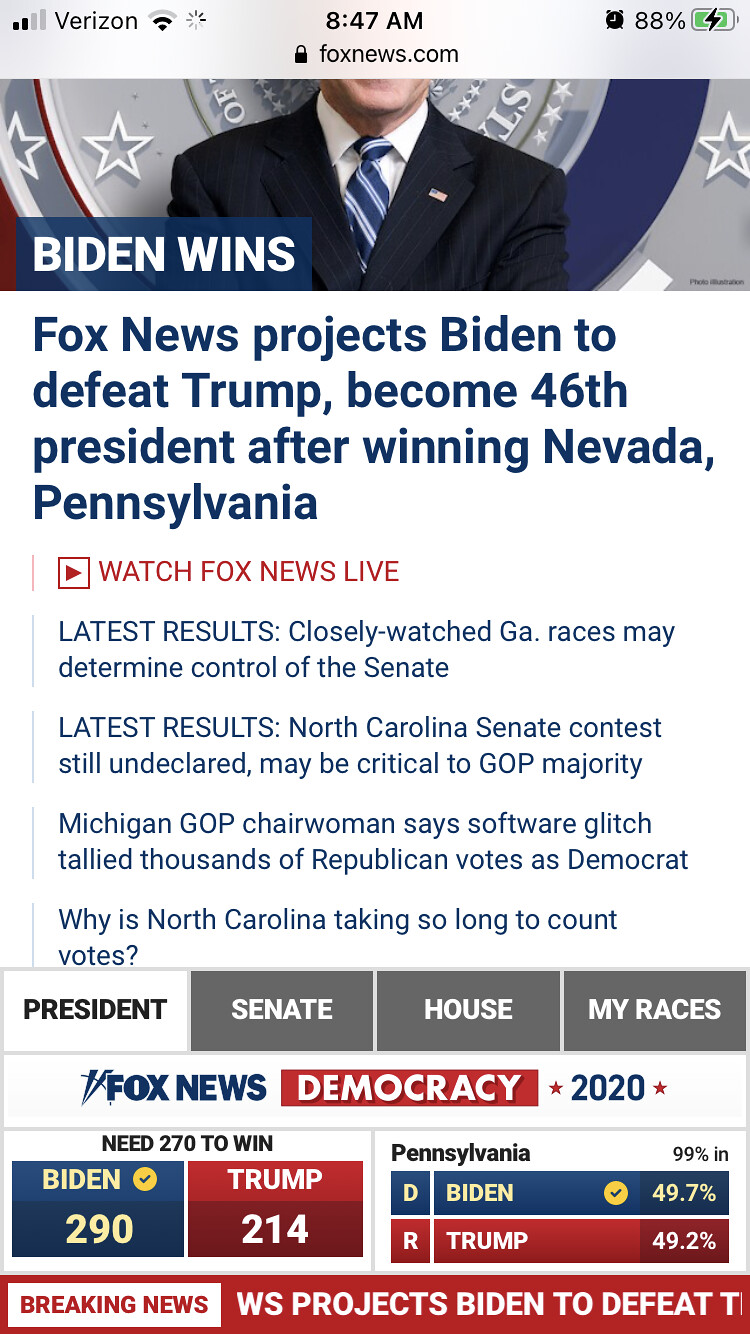The screenshot captures a cell phone display showing a news article from Fox News. At the top left corner of the screen, it indicates the carrier "Verizon" along with the time "8:47 AM." The icons show the device is connected to the internet, an alarm is set, it is currently being charged at 88%, and a padlock symbol next to "foxnews.com" suggests the webpage is secured. The displayed page is cut off mid-scroll, partially showing the bottom portion of a photo likely of Joe Biden, who is wearing a suit and tie. The headline emphatically reads "Biden Wins: Fox News Projects Biden to Defeat Trump, Become 46th President After Winning Nevada, Pennsylvania," followed by a prompt to "Watch Fox News Live," highlighted in red with a triangular play icon. Below this, a rundown of electoral votes shows Biden with 290 votes compared to Trump's 214. Further details mention "Latest Results," including closely watched races in Georgia that may determine Senate control, an undeclared Senate contest in North Carolina critical for the GOP majority, and issues like a Michigan software glitch miscounting Republican votes as Democratic. The screen effectively captures a significant news update and additional electoral information amidst the 2020 U.S. Presidential Election results.